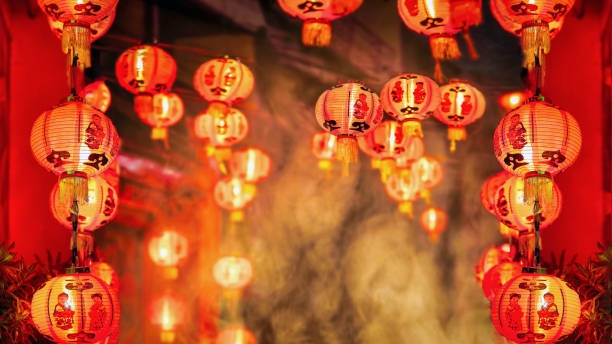The photograph captures a vivid display of Chinese lanterns, likely part of a Chinese New Year's celebration. The scene is set at nighttime, illuminated by a series of red paper lanterns, each resembling an orb or pumpkin shape. These lanterns, adorned with traditional Chinese figurines and dangle tassels, are strung along wires and arranged in vertical lines on both sides of the image. In the foreground, clusters of lanterns stretch from the bottom to the top of the frame, while in the background, a misty or blurry backdrop hints at amorphous buildings or possibly fog. The lanterns serve dual purposes: beautifying the scene and lighting up the surrounding area with their warm red, orange, and yellow hues. The overall ambiance suggests a vibrant, festive atmosphere marked by cultural significance.